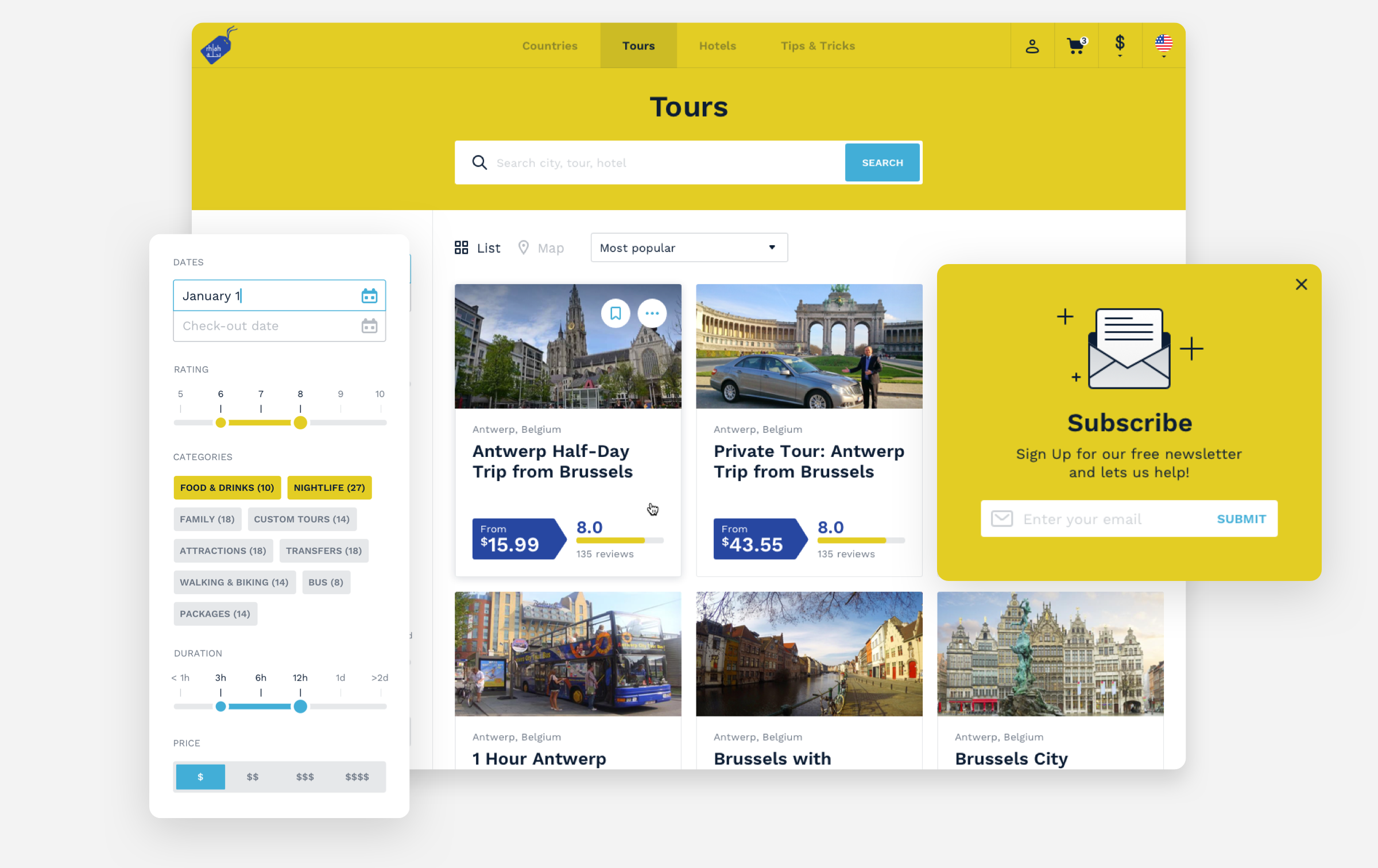The image is a colorful landscape-format screenshot taken from a laptop or desktop computer, depicting a travel website known as Ferula (رِحْلَة). The company's logo features white lettering in both English and Arabic, emblazoned on a blue tag resembling the kind used on luggage. 

At the top of the webpage, various navigation tabs are visible, including options for "Countries," "Tours," "Hotels," and "Tips and Tricks." Additionally, icons at the top right corner represent the user profile, shopping cart, and currency selection.

Prominently displayed in large lettering is the word "Tours," accompanied by a search bar labeled "Search by city, tour, or hotel." The default search setting displays offerings for Antwerp, Belgium, showcasing various tour packages such as "Antwerp Half Day Trip from Brussels."

The user has input January 1st as the check-in date but has not specified a checkout date. They are filtering options to display only those with ratings between six and eight, with a focus on categories such as "Food and Drink" and "Nightlife."